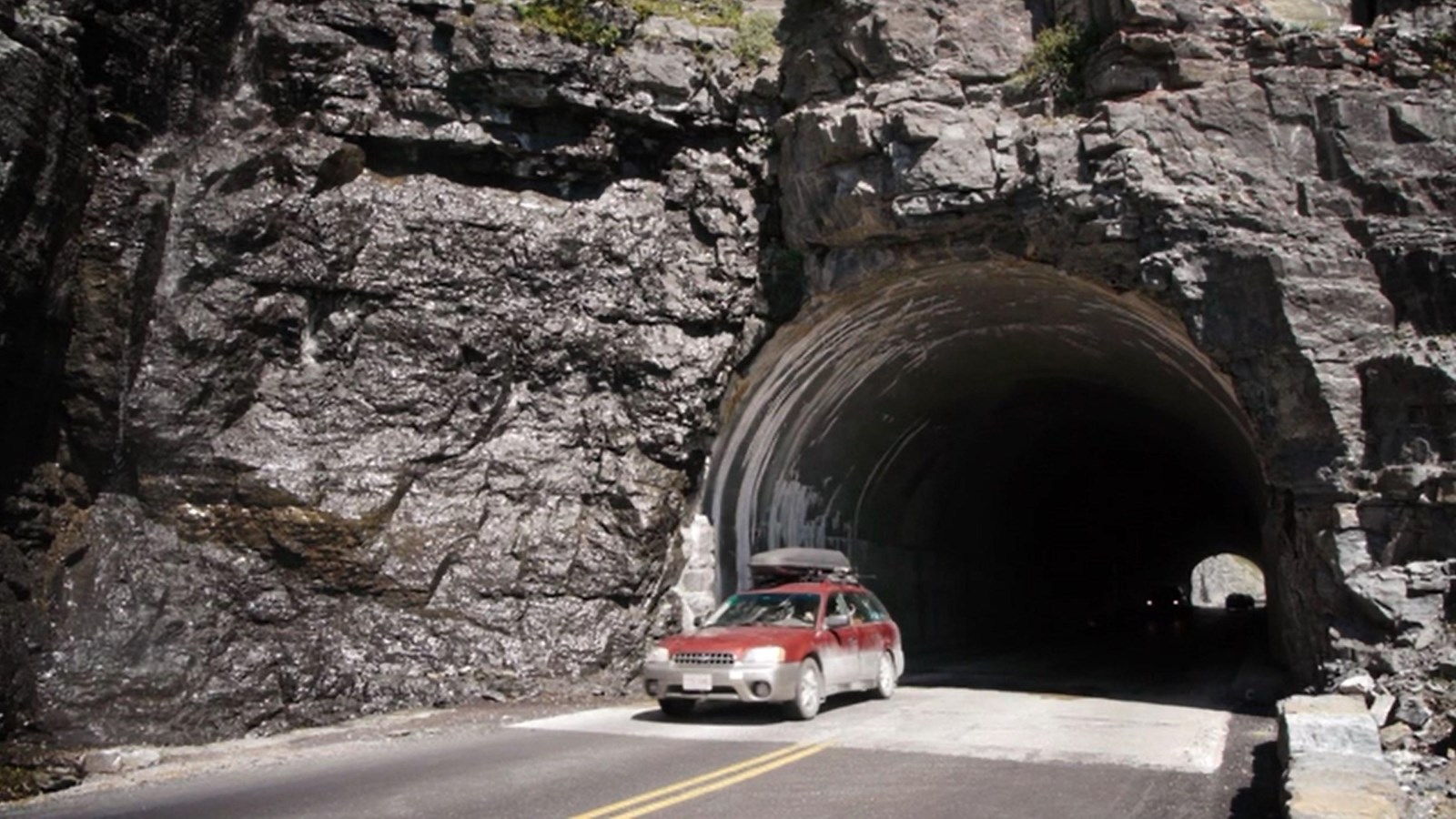The image showcases a stunning outdoor view dominated by a massive rocky mountain composed of dark black stone. A circular tunnel, approximately 100 feet in length, has been meticulously carved through the middle of this solid rock formation. The tunnel's interior is faintly illuminated by sunlight penetrating from the opposite end, where the headlights of another vehicle are visible. Stretching across the bottom of the frame is a two-lane roadway marked with a yellow double line. Emerging prominently from the tunnel and traveling toward the viewer is a red, four-door Subaru crossover with a luggage carrier mounted on its roof. The composition captures the moment as the car, adhering to the right side of the road consistent with European driving conventions, exits the dim tunnel into the open.